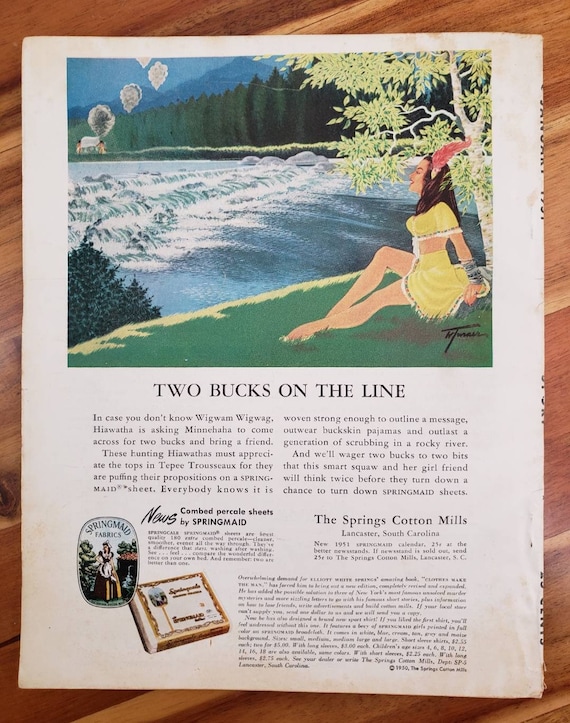This appears to be a page from a 1950s or 60s magazine showcasing an advertisement. At the top is a painting of a woman in a yellow outfit with a white-trimmed crop top and skirt adorned with small dots. She is seated under a tree, smiling with her head arched back, and appears to have a feather in her hair. The setting features a river with white water rapids directly in front of her, and in the distance, there are several trees and subtle images of Native Americans sending smoke signals. Below the painting, the text reads, "Two bucks on the line," followed by several paragraphs beginning with, "In case you don't know wigwam wigwag, Hiawatha is asking Minnehaha to come across for two bucks and bring a friend." The advertisement is promoting Spring Maid sheets, noted to be "woven strong enough to outline a massage." At the bottom of the page is an image of the sheet packaging, featuring a logo with a woman in a long dress set against a backdrop of vegetation. The overall design points to a somewhat crude artistic style common in dated advertisements from that era.